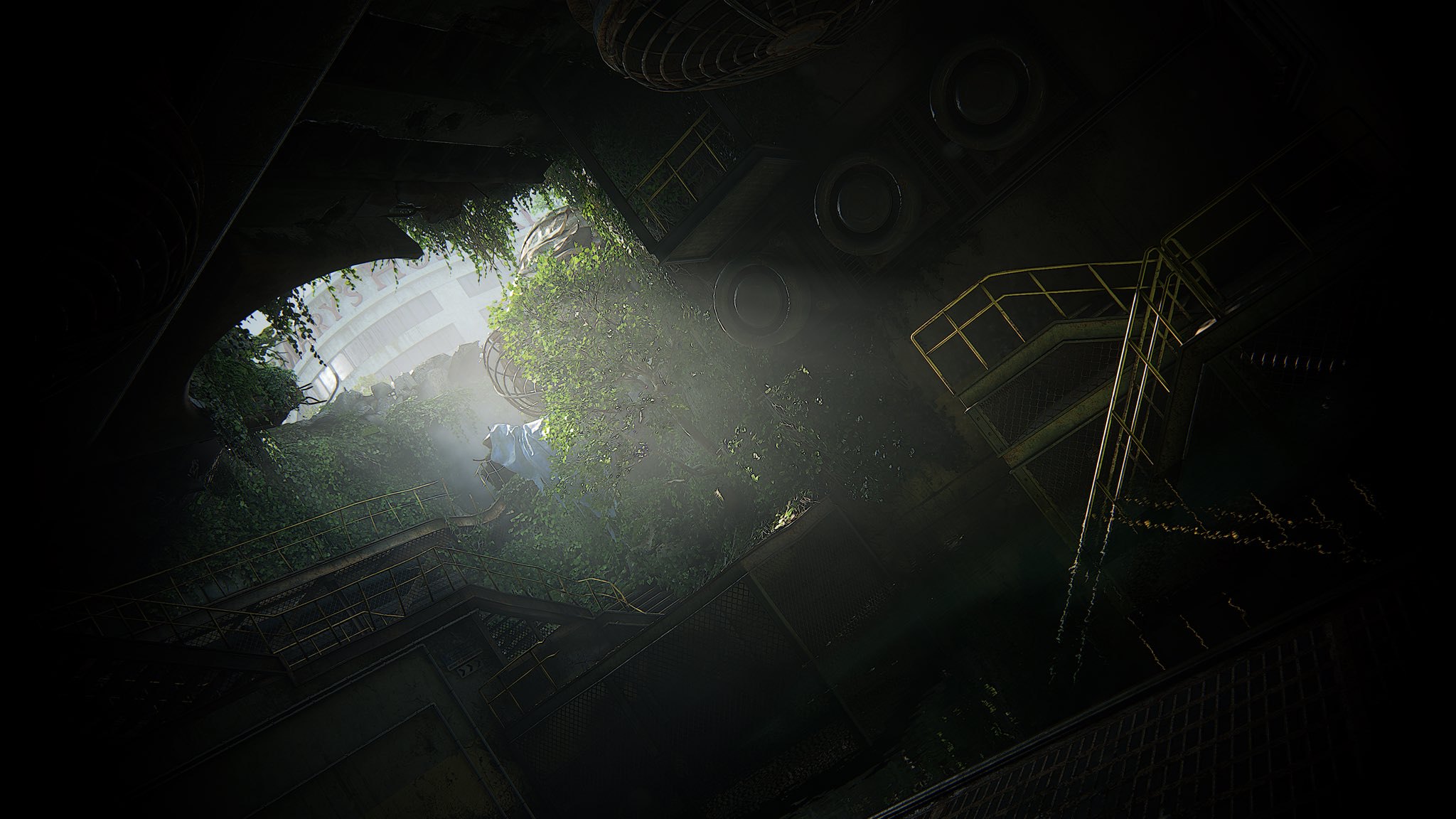The image depicts a detailed digital artwork of an abandoned underground facility or factory setting. It is characterized by a steep set of metal steps that turn a corner onto a platform with metal railings. The facility appears very dark, though beams of sunlight penetrate through an opening, illuminating certain areas. This opening reveals an overgrown exterior with lush greenery, including grass, trees, and vines, giving the sense of a lost, forgotten place that nature has reclaimed. Inside, apart from the steps and railings, there are three circular objects possibly serving as air vents, and some broken-looking balconies. In the distance, through a gap, a modern building with a white facade and red lettering is visible, though the text remains unreadable. A white plastic or paper sheet partially covers a section of the steps or bridge. The digital artwork showcases vivid transitions between light and shadow, highlighting the detailed effort put into its creation.